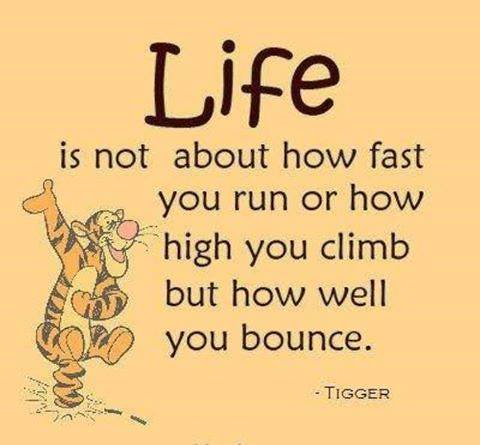The image features a vintage, slightly pixelated color illustration with a peach-orange background. In the center, a bold, fun, cartoony font prominently displays the word "LIFE." Beneath it, a lighter weight font carries the inspirational message: "It's not about how fast you run or how high you climb, but how well you bounce." This quote, attributed to Tigger from Winnie the Pooh, ends with a period. Positioned on the bottom left, Tigger himself is joyfully balancing on his tail with visible impact marks around it. He has a pink nose and a wide, bright pink smile that shows his tongue. His right arm is enthusiastically raised, while his left arm crosses his chest, and both legs are up in the air, emphasizing his lively spirit. The name "Tigger" is capitalized and placed to the right of the quote, completing the whimsical and motivational design.